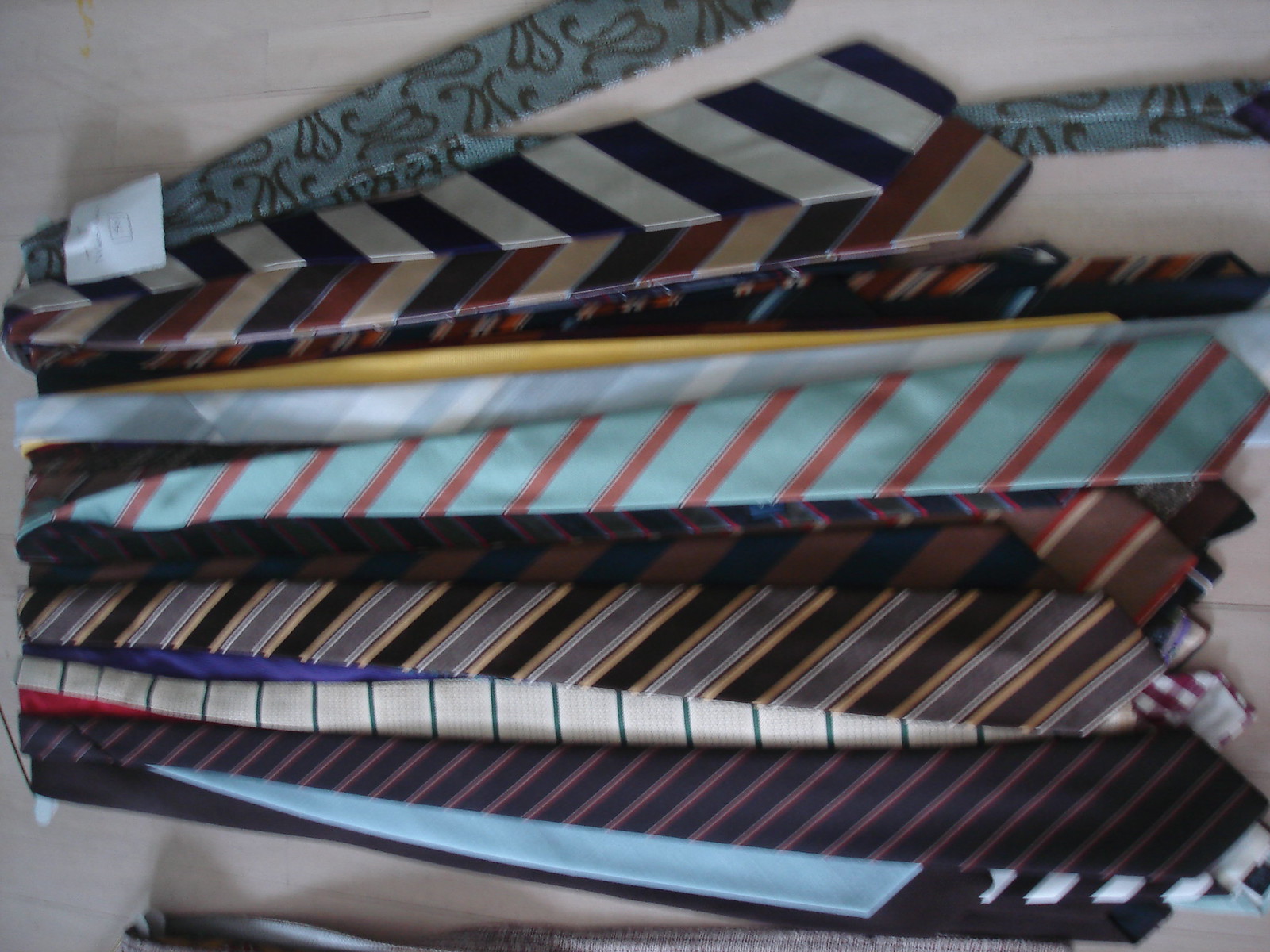The image shows a rather grainy, out-of-focus photograph of numerous neckties draped on a wire hanger, rotated 90 degrees to the left, making the ties appear to be hanging horizontally across the picture. The hanger, which seems cheap and old, is likely against a door or wall, possibly in a bedroom or closet. The collection predominantly features ties with diagonal stripes in various colors and patterns. At the topmost position, there's a light blue tie with a unique paisley design, potentially with a piece of paper pinned to it. Below it are ties with black and white stripes, blue and maroon stripes, and a brown tie with orange, white, and yellow stripes. Further down are more striped ties, including black and gray, blue with orangey-red stripes, and a dark blue tie with red and light blue stripes. There are also solid color ties, such as royal blue, sky blue, and black. The ties vary in color, including shades of blue, brown, and white, and feature combinations like light blue with red stripes, and grey with gold and black stripes. The arrangement is dense, with the ties stacked and draped on each other, creating an impression of abundance and disorder.